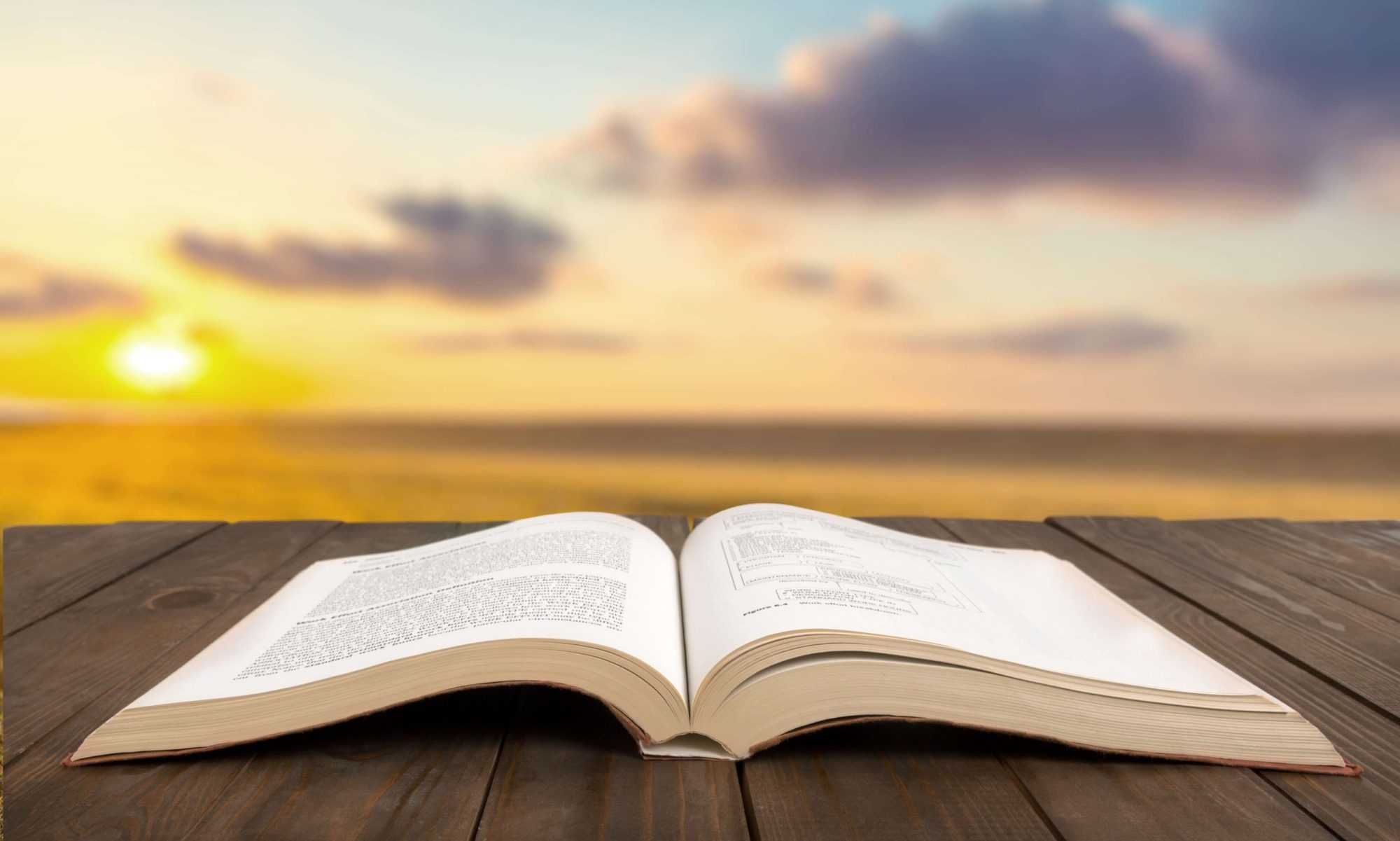The image depicts a close-up view of an open book laid flat on a wooden surface, which could be a picnic table or a dock. The book, with its brown cover and white pages, is open halfway, exposing the slightly curved pages that lean to the left and right, adorned with small black text that is not legible. The wooden surface is composed of darker brown horizontal slats, suggesting a weathered and rustic appearance. The background, though blurred, showcases a stunning horizon with a vast body of water, possibly an ocean or beach. Prominent in the distant background is a glowing yellow sun, likely setting, casting a warm light across the scene. The sky features large clouds with a light reddish-pink hue, adding to the serene and picturesque ambiance of the setting.